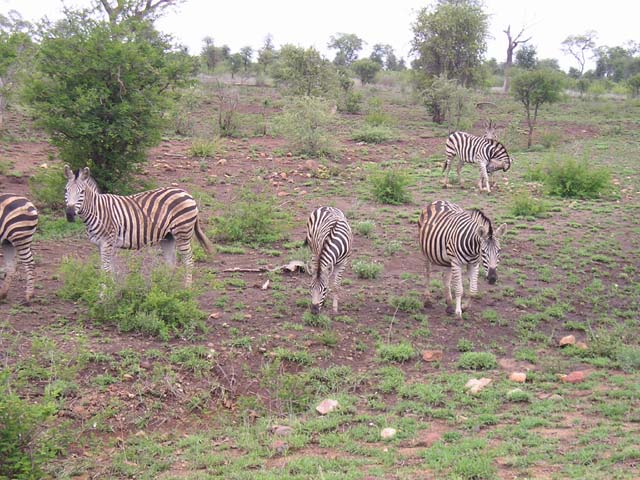This is a detailed, color photograph capturing a group of five zebras in what appears to be a wildlife reservation or a zoo. The scene is set on stony, rocky ground interspersed with clumps of grass, shrubs, and some brownish or white objects that could be stones or mushrooms. In the foreground to the left, only the hind legs of one zebra are visible. Next to it, a slightly dirty zebra is fully visible and faces the camera while standing to the left. The central zebra has its head down, feeding on grass, facing slightly toward the camera. To its right, another zebra looks poised to start eating grass as well, while further back, one zebra partially obscures another who is almost hidden. The partially obscured zebra's head is turned slightly downwards, facing right. The background features larger shrubs and tall trees with green leaves, set against a greyish-white overcast sky, adding depth and a sense of the environment to the image.